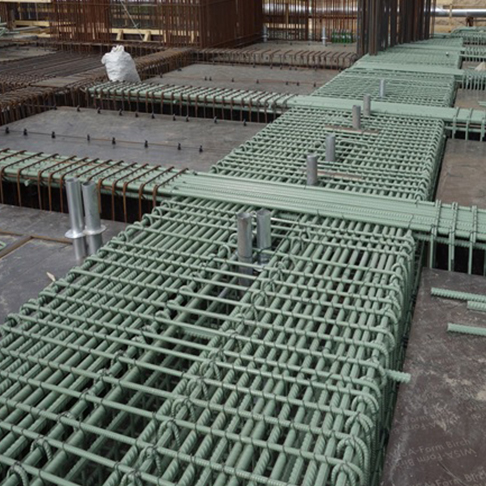The image depicts an industrial construction site characterized by a bronze-tinted ground with green elements, possibly aged copper. Central to the scene is an array of metal pipes and wires intricately intertwined, resembling a woven structure. From a top-down perspective, you can see rows of rebars extending backward and horizontally, creating a grid-like pattern. Silver smokestacks rise amidst these structures, lending a vertical dimension. In the background, concrete is being poured, and more pipes and wires are being laid down, forming the foundations of a budding industrial building. To the top left, a solitary trash bag lies amidst the meticulous chaos, hinting at the bustling activity on-site.